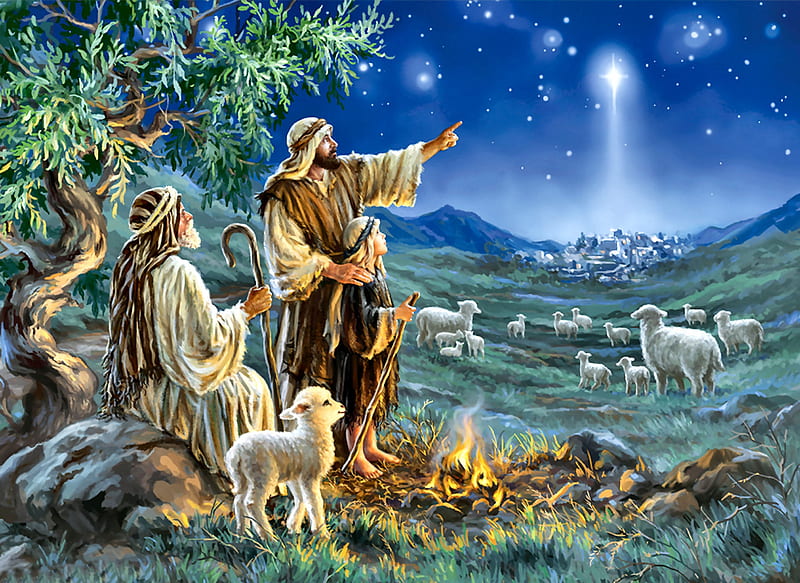The painting-like digital illustration depicts a serene Biblical scene under a starry night sky, with particular emphasis on the Star of Bethlehem glowing prominently just off-center to the right. Set against a backdrop of low hills and mountains, and with a distant view of an ancient city nestled in a valley, presumed to be Bethlehem with its clustered white buildings, the scene unfolds in a wide, vertical rectangle. 

In the foreground, a group of shepherds is gathered around a small campfire under a large tree. The oldest shepherd, a man with a white beard, draped in a white robe and holding a staff, sits on a rock next to a lamb. He is surrounded by numerous other sheep, both grown and young. Standing beside him is a younger man with a brown beard, wearing traditional head drapery secured with a band, hand resting on the shoulder of a young boy holding a walking stick. This younger man is pointing towards the bright star, offering guidance to the boy who looks up in awe. The lush grassy field stretches from the shepherds to the city, dotted with other sheep grazing, creating a pastoral and peaceful atmosphere. The scene is imbued with warmth and wonder, capturing the divine night thought to herald the birth of Jesus.